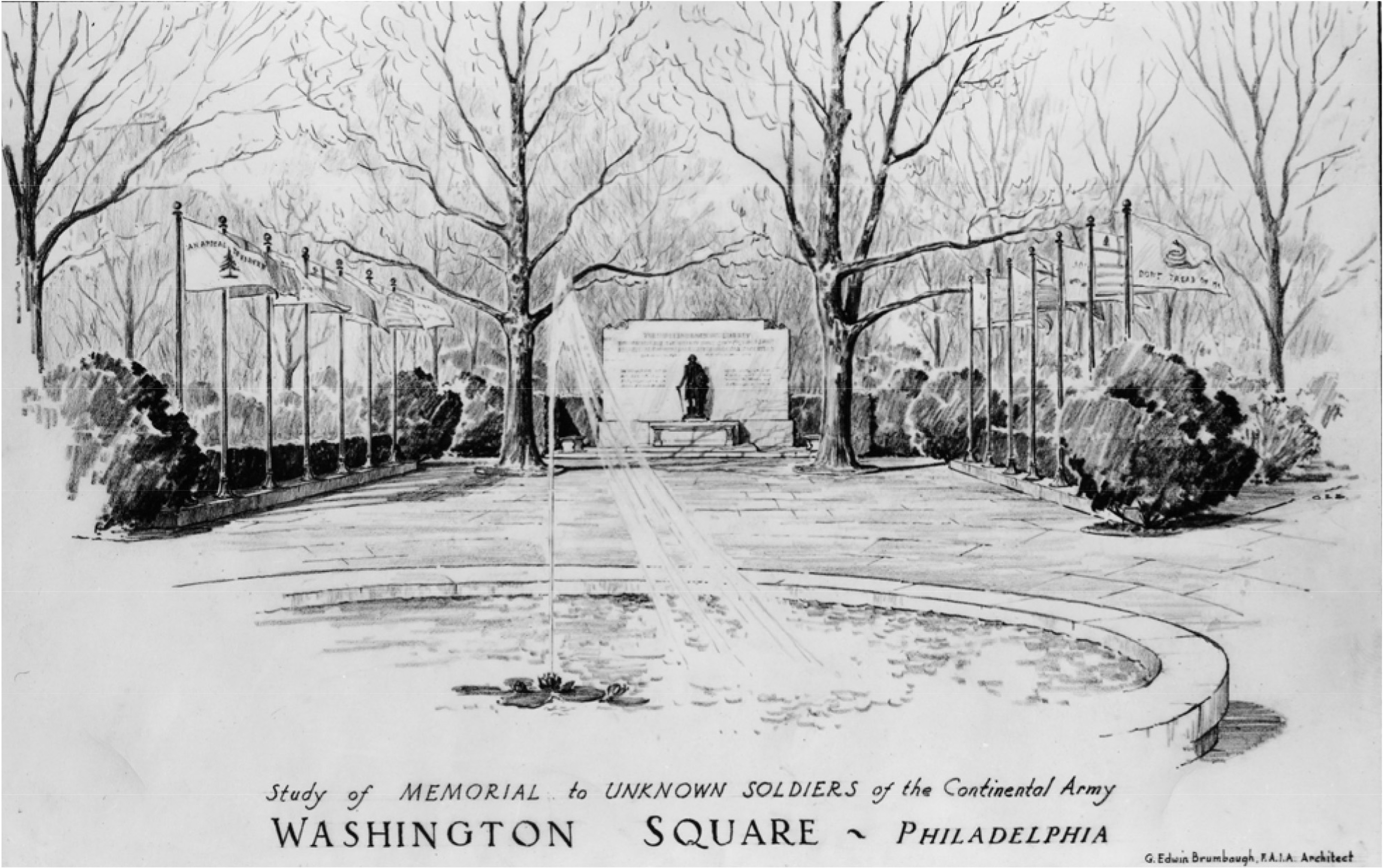This black and white drawing, set in a square format with an off-white background, captures an outdoor scene in Washington Square, Philadelphia. The image depicts a "Study of Memorial to Unknown Soldiers of the Continental Army" as noted in text at the bottom, along with the source "G. Edwin Brown Book, K.A.I.A. Architect" in the bottom right corner. The foreground features a low-lying, round fountain with white water elegantly shooting out of it. The area is blanketed with leafless trees and bushes, accentuating a winter-like atmosphere. Adorning the scene, rows of curling flags line a paved walkway leading towards a central marble memorial plaque and statue. Prominent among the flags are the "Don't Tread on Me" flag and another with a pine tree, representing different American colonies. The walkway is flanked by two large, barren trees, further enhancing the somber and reflective mood of the memorial dedication.